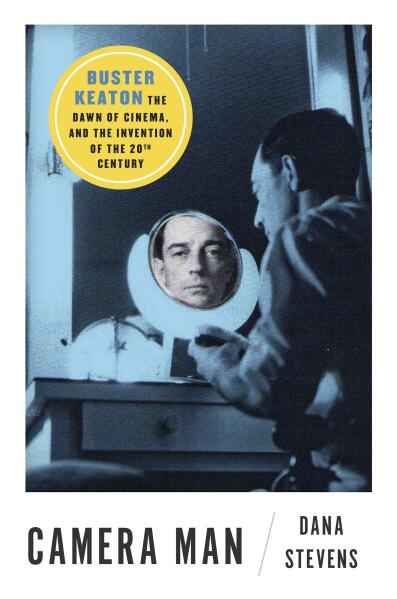The image resembles a movie poster or book cover, dominated by a dark gray palette with subtle bluish lighting. In the upper left corner, a round, yellow stamp-like logo reads, "Buster Keaton: The Dawn of Cinema and the Invention of the 20th Century." Central to the composition is a man seated at a desk, his body turned away from the viewer. The desk, light-colored and featuring a drawer, supports a round mirror positioned prominently in the middle of the image. The man’s profile is partially visible, but his face is fully reflected in the mirror, showing dark features, black hair, and pallid skin. At the bottom of the image, in dark gray font, are the words "Cameraman / Dana Stevens."